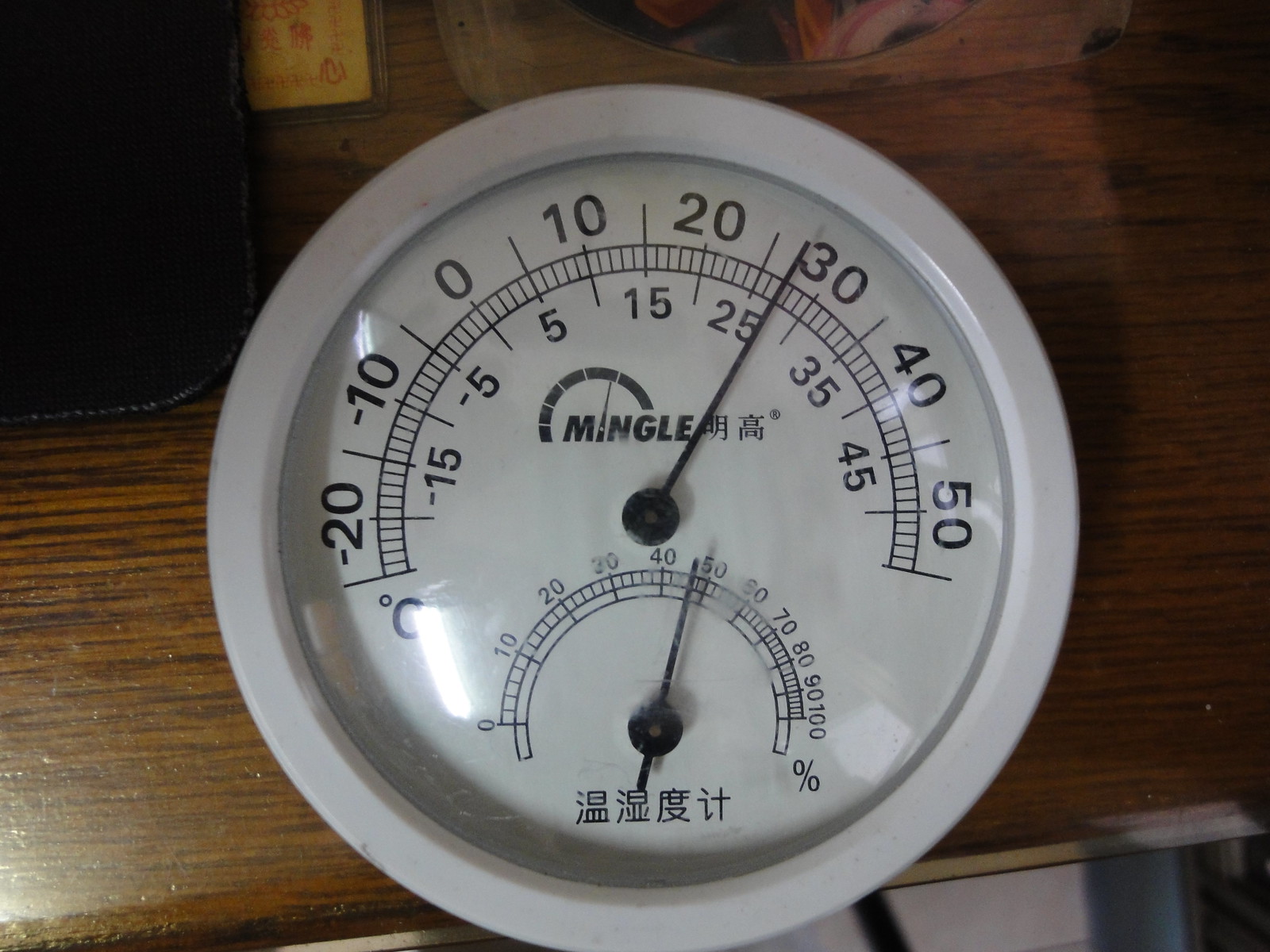The image presents a detailed view of a dual gauge dial. The upper section of the dial displays large numbers ranging from -20 to +60, and beneath this, there is a secondary scale ranging from -10 to +50. Positioned to the left of the indicator hand on the upper gauge is the word "MINGLE." Currently, the indicator hand is pointing to approximately 27 on this upper scale. 

Below the upper gauge, there is a smaller gauge marked from 0 to 100, which includes a percentage sign (%). The indicator on this lower gauge is pointing at around 47. Beneath this smaller gauge, text is visible, written in either Japanese or Chinese characters, further adding to the complexity and specificity of the dial.